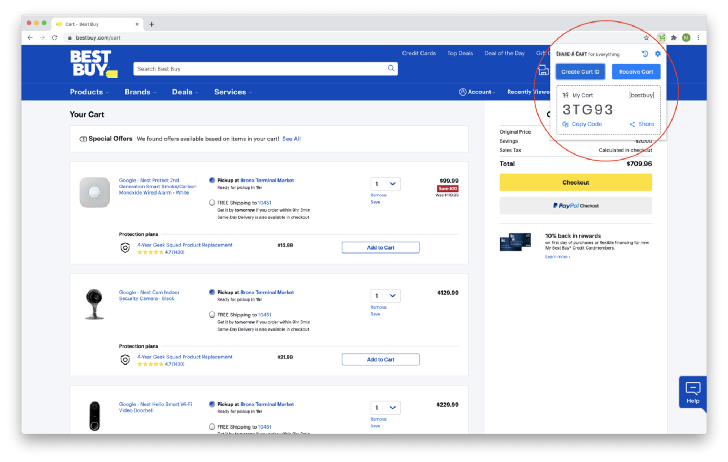This image captures a detailed screenshot of the Best Buy website's shopping cart page. At the top of the page, a distinctive blue banner features the white "Best Buy" text and their iconic yellow price tag logo. On the top right, there's a prominent search bar, accompanied by several drop-down menus labeled "Products," "Brands," "Deals," and "Services."

Highlighted in a red circle on the right is a mysterious drop-down box, featuring text that appears to be in a foreign language. This element obscures part of the right-hand side of the page, possibly serving as some sort of verification box.

On the left-hand side, a section titled "Your Cart" outlines special offers available. It mentions, "We found offers available based on items in your cart," with an actionable "See All" button below. Beneath this, three tiny product images are displayed, which appear to be a router, a mounted camera, and possibly a speaker, though the exact details are indistinct.

Monetary details are shown on the right side of the page. While the breakdown of the original price and taxes is not visible, the total cart amount is clearly listed at $709.96. Below this total, a prominent yellow "Checkout" button and a supplementary "PayPal Checkout" button are displayed, providing convenient checkout options for the user.